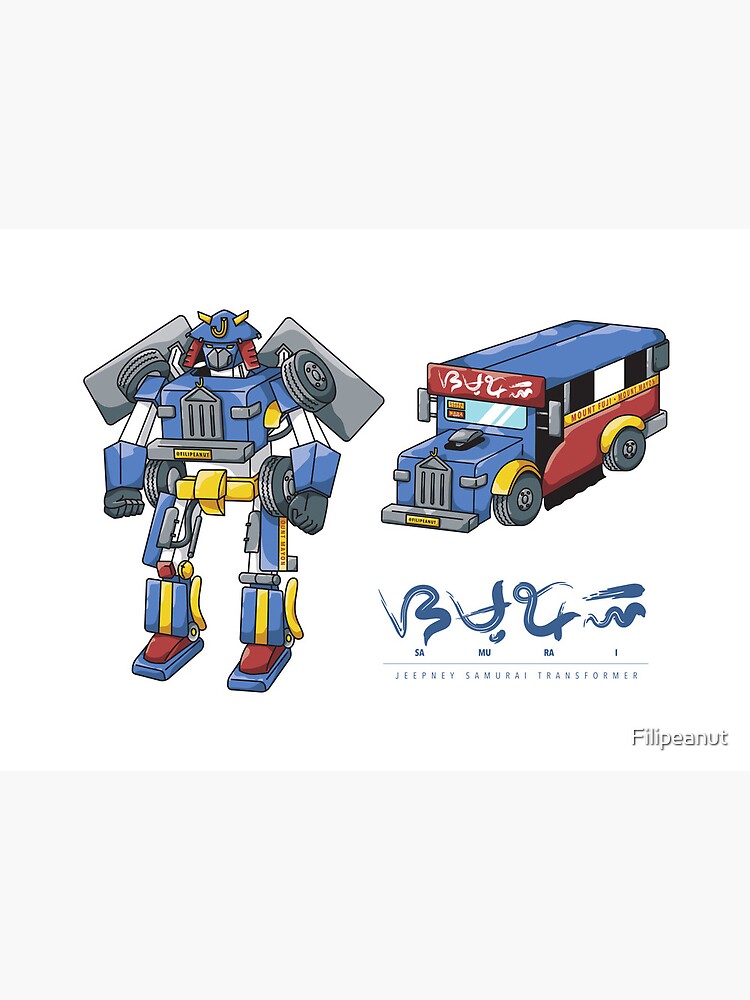The image is a landscape-oriented digital sketch featuring an action-packed, transformer-like robot that converts into a bus, infused with an Asian, specifically Japanese, aesthetic. On the left side, the robot, standing in a dynamic pose, is predominantly blue and white with striking red and yellow accents. Its design cleverly integrates bus components: wheels on its shoulders and hips, panels, and a chest formed by the front of the bus, complete with a license plate. The robot dons a Viking-like helmet with a “J” on it, enhancing its samurai persona.

On the right side, the bus, depicted in the same vibrant cartoon style, showcases a blue roof and front, with raspberry red and yellow side panels, and gray wheels. Prominently displayed on the side of the bus is "Mt. Fuji" along with Japanese characters, matching the samurai symbols found on the robot. The bus’s flat roof and the red sign with white writing above the driver's window add to its unique design.

At the bottom, in elegant Japanese script and small blue English font, is the title "Jeepney Samurai Transformer." Below these, a watermark reads "Filipinot" in white with a black outline, suggesting the artist or designer's signature. The entire composition is set against a clean, white background, making the vibrant colors and intricate details of the transformer and bus stand out.